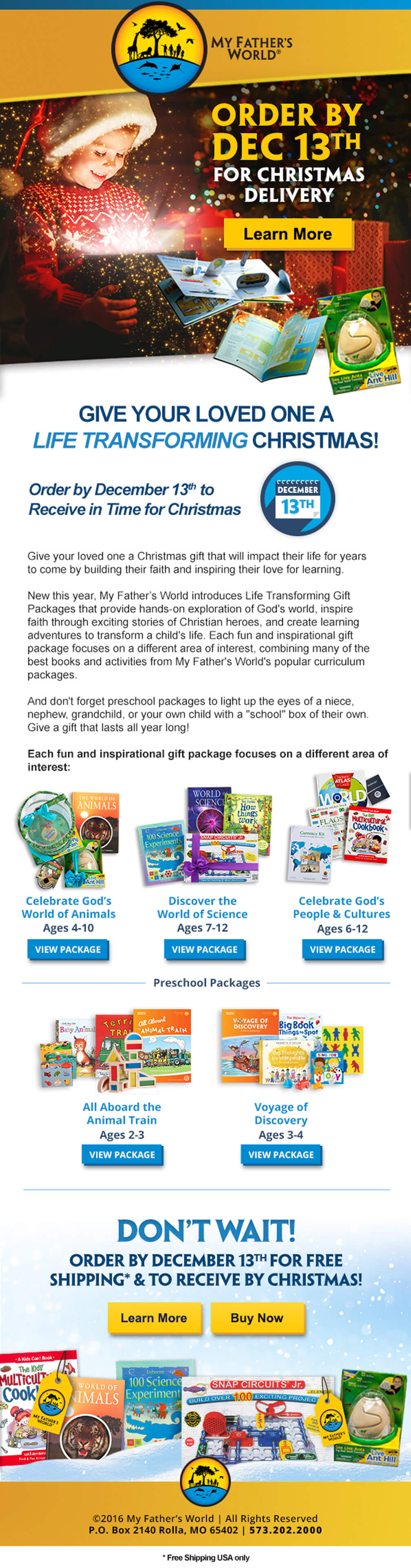This is a website screenshot for My Father's World. At the top of the page, there's a logo featuring African animals and a tree within a circular emblem. Below the logo, a young girl wearing a Santa Claus hat is pictured. Superimposed on her image, in yellow text, it reads "Order by December 13th" and in white text "for Christmas delivery." Directly beneath this, there is a yellow button labeled "Learn More." Scattered around the girl's image are various children's books.

Further down, a blue heading reads, "Give your loved one a life-transforming gift." Underneath, smaller blue text states, "Order by December 13th to receive in time for Christmas," accompanied by a circular icon depicting a December 13th calendar. The next section elaborates on the gift offerings, saying, "Give your loved one a Christmas gift that will impact their life for years to come by building their faith and inspiring their love for learning." It announces new life-transforming gift packages introduced by My Father's World, which offer hands-on exploration of God's world, inspire faith with Christian hero stories, and create learning adventures designed to have a lasting impact on a child's life. Each package focuses on a unique area of interest, combining a selection of the best books and activities from My Father's World's popular curriculum packages.